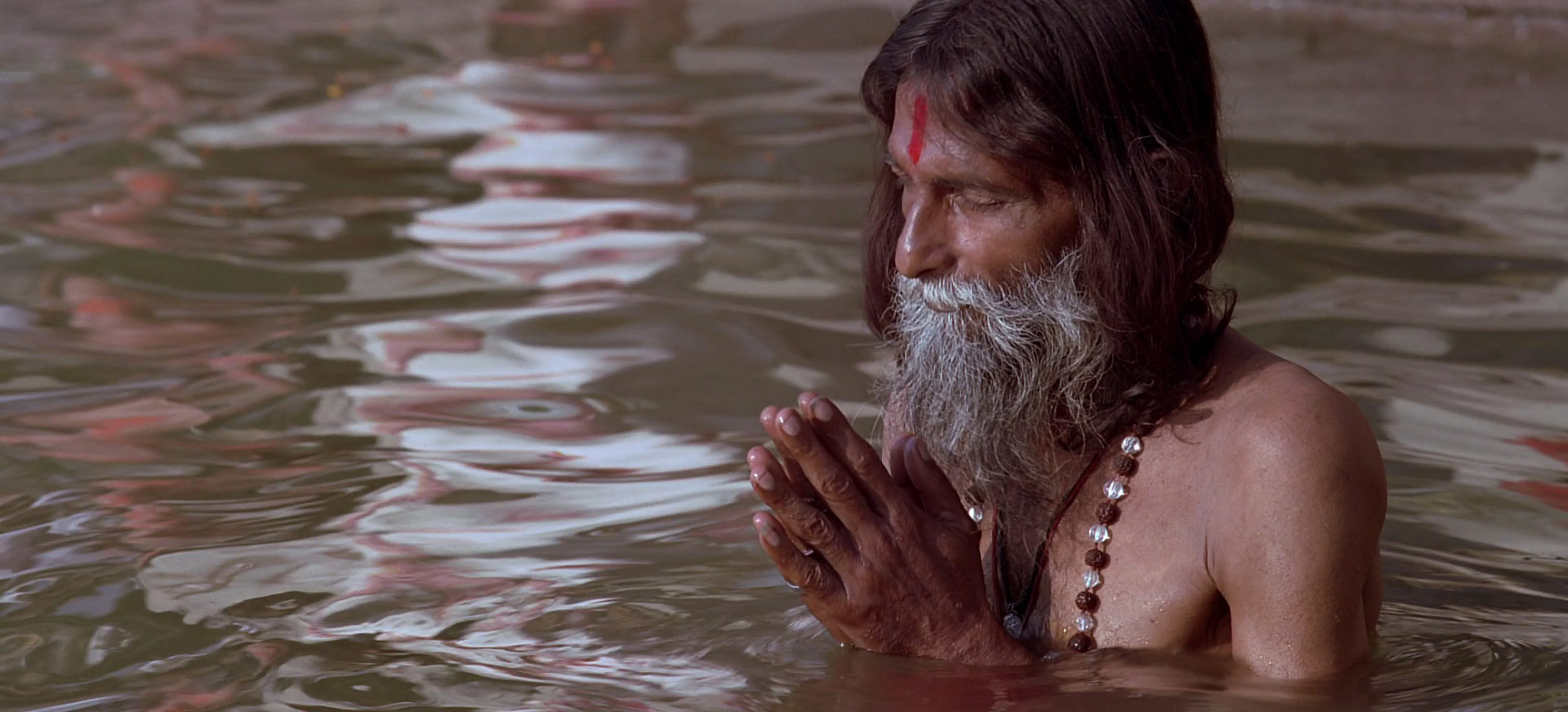In the color photograph, styled in representational realism, an older man with dark skin, long, wavy brown hair, and a gray beard stands in a reflective body of water. Positioned towards the right of the center, the photo captures him from the middle of his head to his chest, the rest of his body submerged. His hands are clasped in front of his mouth in a prayerful manner, with his eyes closed and a red vertical paint stripe on his forehead, suggesting a religious significance. He wears no upper garments, but a beaded necklace in shades of brown and white adorns his neck. The water around him, a murky greenish-brown color, reflects light, possibly from a distant source or nearby people in white clothing, although the water's ripples obscure a clear reflection.